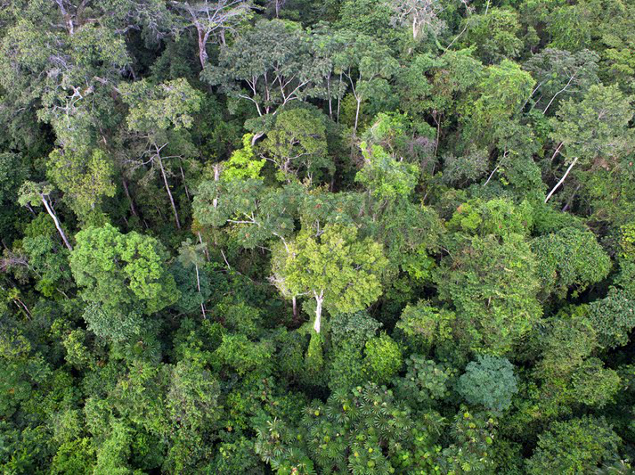An aerial image reveals a dense, lush forest canopy resembling a jungle. The verdant landscape is characterized by a mix of cypress and mangrove-like trees, their light-colored trunks and limbs adorned with Spanish moss. The treetops present a medley of green shades, from bright lime and new growth to more subdued tones, creating a rich tapestry of colors. The canopy is so thick that the ground, dirt, rocks, and any wildlife are completely obscured. The trees have various rounded shapes, akin to miniature broccolis, contributing to the forest's full and bulbous appearance. The scene is brightly illuminated, enhancing the intricate details and vibrant hues of this natural setting. In parts of the dense foliage, there are clusters of bushes with small, round, apple-like formations, adding even more texture to the vivid landscape.